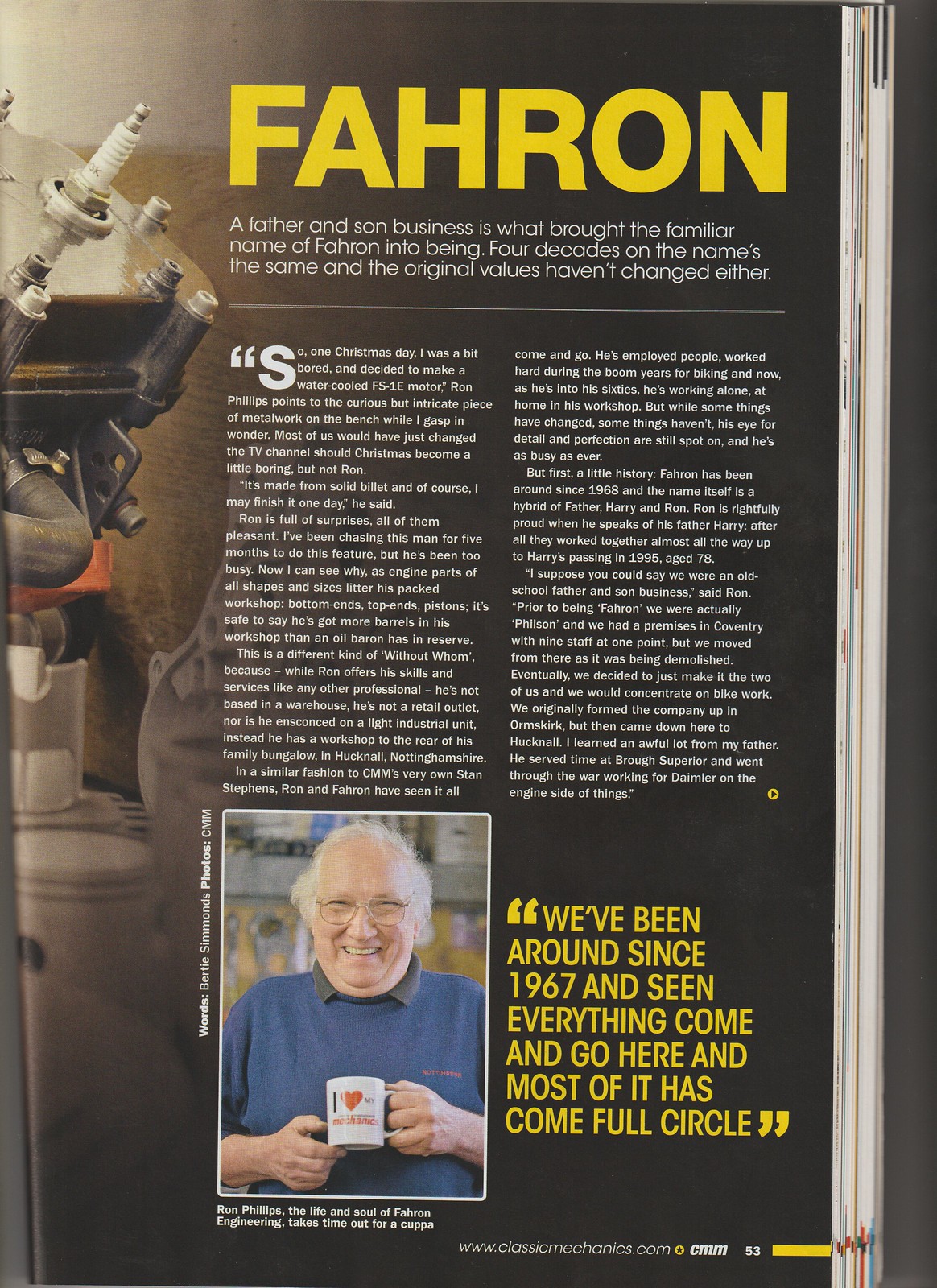The image is a color advertisement or a magazine page with a dark background transitioning from black to brown. At the top, in bold yellow letters, is the word "FAHRON." Beneath that, there are three lines of small white text stating, "A father and son business is what brought the familiar name of Farron into being. Four decades on, the name's the same and the original values haven't changed either." The bulk of the page contains two columns of small white text that are not easily readable. On the left side, partially seen, is a tan and silver machine, possibly with a spark plug. At the bottom of the page is a section with a photograph of an older man with a receding hairline, white hair, and glasses. He is smiling and holding a white mug, dressed in a blue vest, t-shirt, or sweater. Next to his image, a quote in large yellow letters reads, "We've been around since 1967 and seen everything come and go here. Most of it has come full circle."